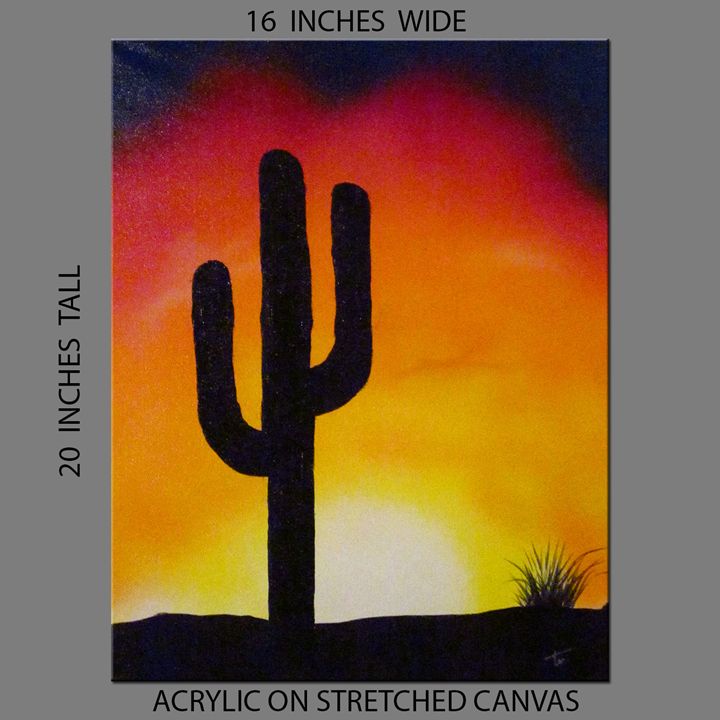The acrylic painting, presented on stretched canvas, showcases the silhouette of a saguaro cactus at sunset. The scene is backlit by a glowing white orb of the sun nestled just above the horizon. This light source transitions through a spectrum of warm colors—yellows and light oranges near the bottom, fading into darker oranges, and culminating in red and eventually black at the top. Complementing the central cactus silhouette, the ground beneath it is also rendered in solid black, with a small, bushy plant adding detail to the right. The entire image is framed by a medium-toned gray border. On the left border, from bottom to top, black text reads "20 inches tall." At the top edge, similar text states "16 inches wide," while the bottom denotes "acrylic on stretched canvas." The image is rich in color and high in clarity, capturing the natural lighting of a vivid sunset.